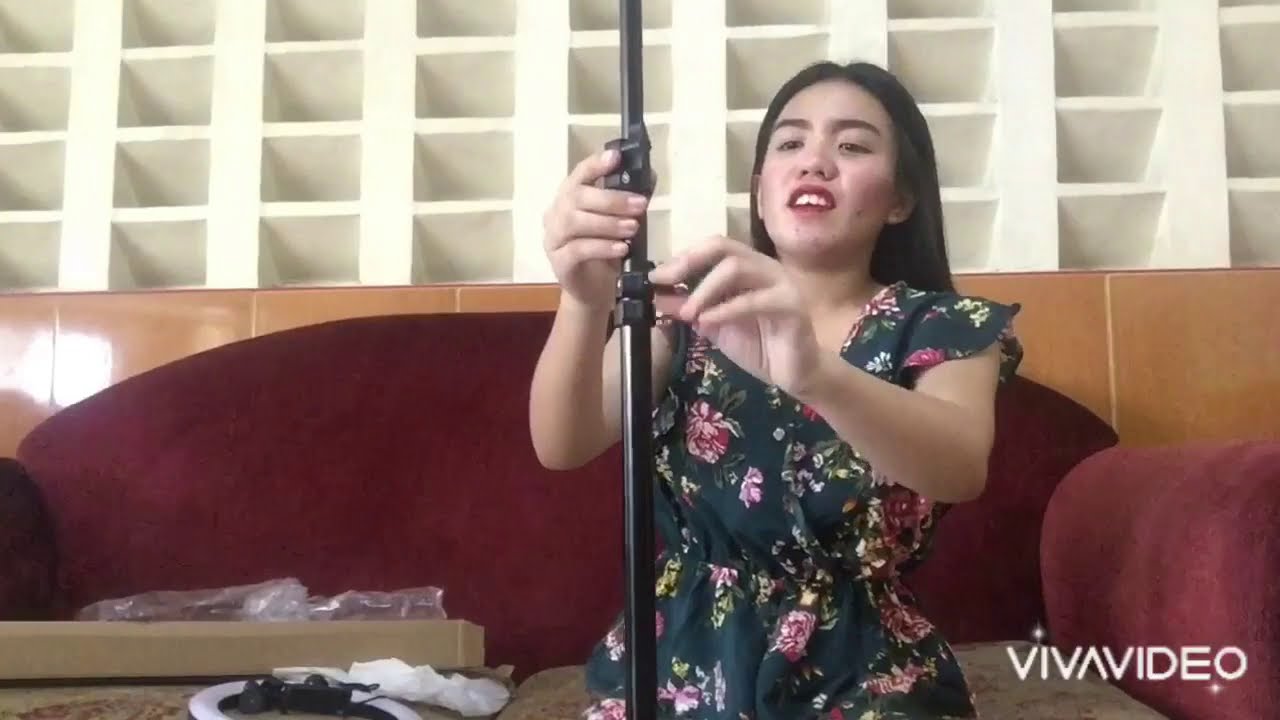In this detailed color photograph, an Asian woman with long black hair is seated on a velvety dark red couch, intent on assembling a black metal pole from a cardboard box beside her on the couch. The couch itself has brown cushions. She is wearing a sleeveless dark green dress adorned with a floral pattern in yellow, pink, and rose hues. Her lips are accentuated by heavy lipstick, and she appears to be wearing significant makeup, with her mouth slightly open in concentration. Scattered around the open box are plastic bags and other black plastic components that accompany the pole she is setting up. Behind the couch, there is brown shelving, and further behind is a wall with patterned square cubby holes. Among the items in the room is a circular object containing black elements and a white, crumpled piece of paper or napkin on the left side. In the bottom right corner of the image, the watermark "Viva Video" is displayed, surrounded by small stars.